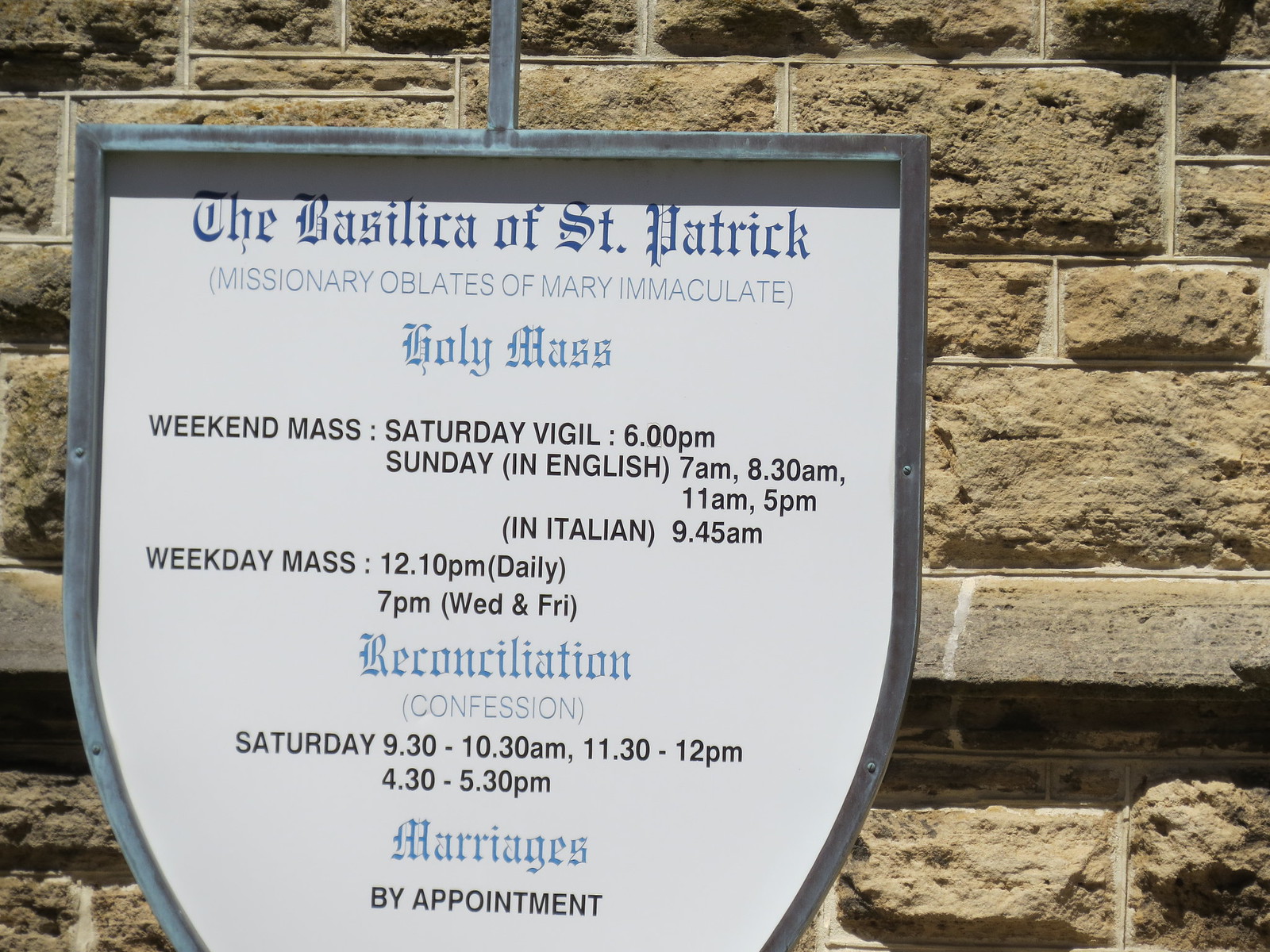The image showcases a detailed sign posted on the exterior of a building that closely resembles a brick structure but is actually made of stone siding. The sign itself has the shape of a shield and features a white background with a metal frame. At the top, it reads "The Basilica of St. Patrick, Missionary Oblates of Mary Immaculate." The sign provides an extensive schedule of Holy Masses and services offered by the church.

The Weekend Mass schedule includes a Saturday Vigil at 6 PM, and Sunday Masses in English at 7 AM, 8:30 AM, 11 AM, and 5 PM, with an additional Mass in Italian at 9:45 AM. Weekday Mass is held daily at 12:10 PM, with extra services on Wednesday and Friday at 7 PM. The sign also details the times for Reconciliation and Confession: Saturdays from 9:30 to 10:30 AM, 11:30 AM to Noon, and 4:30 to 5:30 PM. It notes at the bottom that marriages are by appointment only.

The text on the sign is a mix of an old-style font for headings and regular, everyday font for dates and times. This sign serves as an informative guide to the church's weekly activities and is prominently displayed on the side of the building.